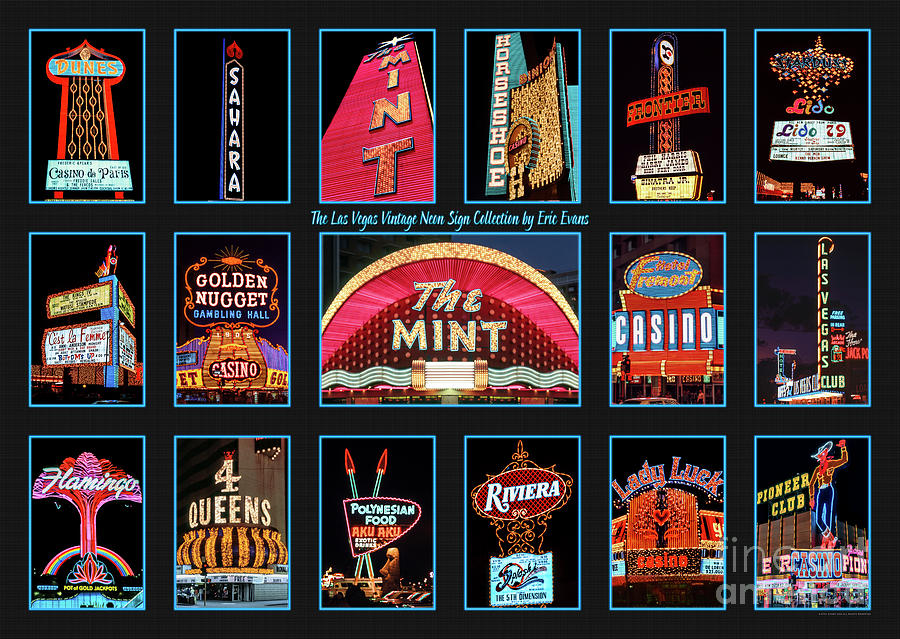This image features a meticulously curated collage titled "Las Vegas Vintage Neon Sign Collection." Set against a black background, it comprises eighteen iconic Las Vegas neon signs, arranged in three rows of six. Each photograph is bordered in light blue and showcases a different casino sign. The top row includes the Dunes, Sahara, Mint, Horseshoe, Frontier, and Lido signs. The middle row features C'est La Femme, Golden Nugget, a second Mint, Fremont Casino, Las Vegas Club, and Flamingo signs, though some are harder to read from a distance. The bottom row displays signs for Flamingo, Four Queens, Polynesian Food, Aku Aku, Riviera, Lady Luck Casino, and Pioneer Club Casino. This collection pays homage to the vibrant history of Las Vegas's nightlife through its vintage neon artistry.